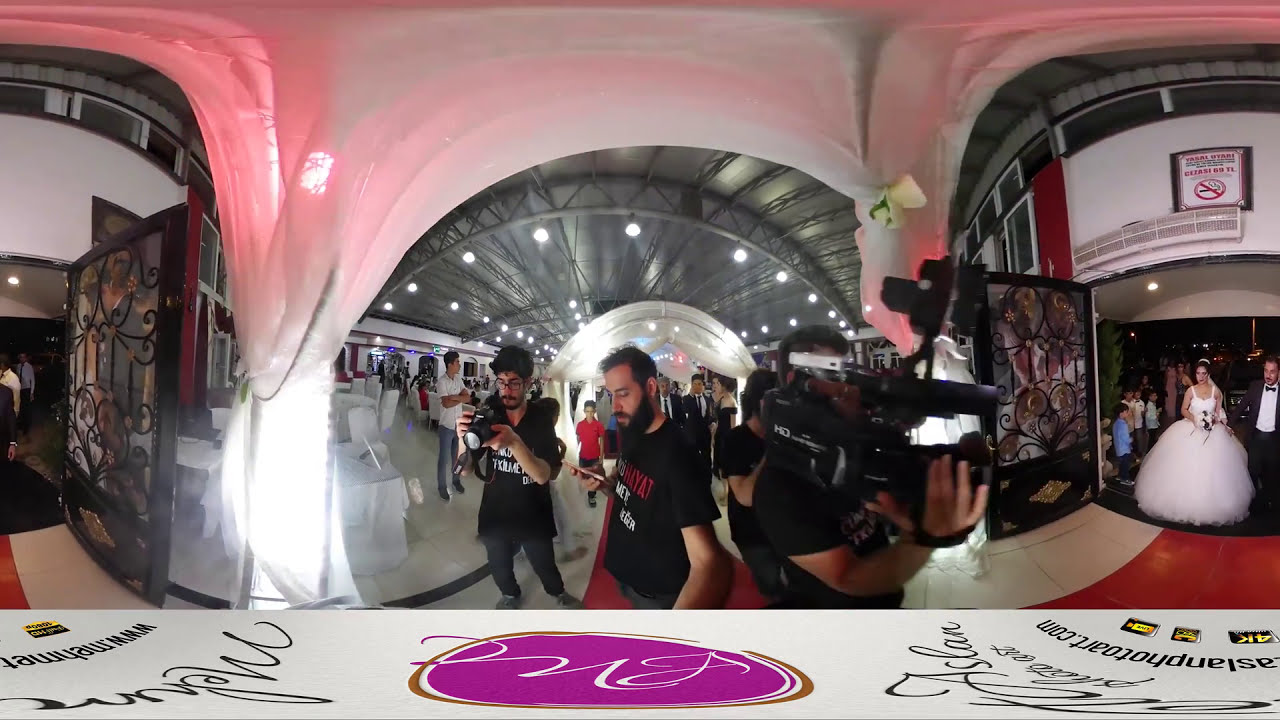This detailed panoramic photograph captures a lively wedding scene set within what appears to be an indoor venue. The image's most prominent feature is a trio of men dressed in black t-shirts, presumably as part of the wedding's photography team. The man on the right holds a large professional video camera, the man on the left wields a standard handheld professional camera, and the central figure captures moments on a cell phone. Each shirt bears red and white text that isn't entirely legible but adds a uniform element to their appearance. Behind them stands another man in similar attire, slightly obscured from full view.

To the right of this group, a couple stands poised, ready to be photographed, signifying that it is their wedding day. The bride is adorned in a classic white wedding gown, and the groom is dressed in a tuxedo with a white undershirt. They seem prepared to walk down a red carpet that extends in front of them, leading to an arched, mirrored hallway, indicative of a grand entrance.

The venue's intricate details include a black, arched ceiling with exposed rafters, white walls punctuated by a vent, a no-smoking sign above the door, and a somewhat eclectic floor pattern of red and white. Behind the main subjects, there is a mix of attendees: a little boy in a red shirt and black shorts, a man in a white shirt and blue jeans standing with crossed arms, and tables adorned with white tablecloths and chairs.

The image's upper portion is tinged with a pink hue, adding a whimsical touch. The text on the banner or possibly an upside-down table provides a mixture of cursive and block fonts, with phrases such as "live" or "love" appearing subtly. This wedding scene is a vibrant tapestry of people, colors, and textures, immortalized through the keen eyes (and lenses) of the photographers.